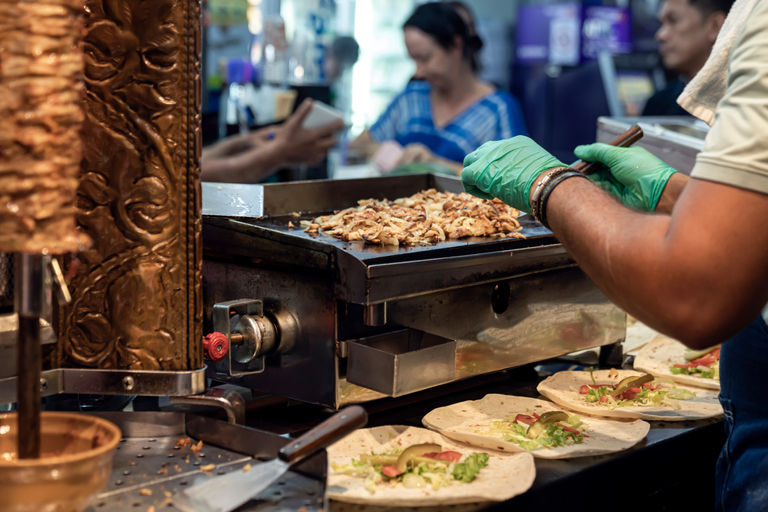The photograph captures the bustling kitchen area of a food shop, where the main focus is a person cooking on a raised black metal griddle. The cook's hands, donned in green gloves, maneuver a spatula over pieces of chicken that exhibit white and brown tinges as they cook. Below the griddle, a row of tortillas lined with avocado, tomato, and possibly onion awaits the addition of the chicken. The cook, whose face is not visible, shows only a sliver of their body to the right side of the image.

On the far left, there's a vertical spit, likely a shawarma rotisserie, showcasing layers of rotating meat, with a copper-colored splatter guard behind it. Surrounding the kitchen area, the shop extends into a blurry yet discernible customer zone. Directly behind the counter, part of a man’s face is visible, while a young woman, dressed in a blue plaid top, stands to the left, possibly writing something down with a pen on a pad.

Adding to the liveliness, other metallic cooking implements and structures can be seen scattered around. The background adds depth, resembling a convenience store with indistinct people moving about, including a man standing behind a woman at the counter. Overall, the photograph vividly portrays a dynamic, busy food preparation scene within the shop.